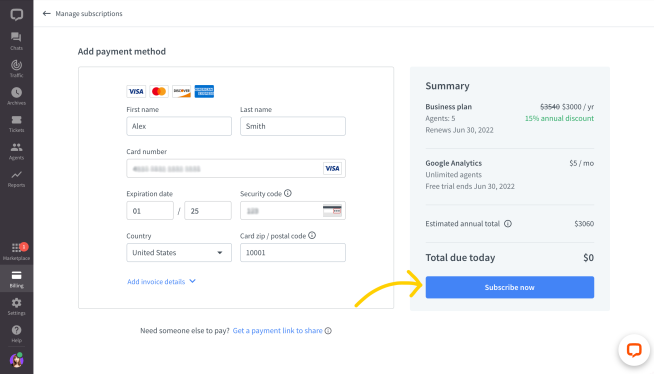The image displays a payment page, characterized by a detailed and user-oriented interface.

**Left Panel:**
- The left-hand sidebar features a column of small icons representing different functionalities, albeit somewhat difficult to read. These icons include:
  - Chats
  - Accounts
  - Tickets
  - Agents
  - Settings
- Additionally, there’s a symbolic representation of a person, indicating either a user profile or account settings.

**Main Center Panel:**
- The central section prominently displays the header "Add Payment Method."
- Beneath this header are logos of four major credit card providers: Visa, MasterCard, Discover, and American Express.
- The first input line contains two text boxes labeled "First Name" and "Last Name," filled with sample data: Alex Smith.
- The next input line, "Card Number," displays a sample Visa card number.
- Following that, there is an input line for "Expiration Date" (noted as 01/25) and "Security Code," which is blurred out for privacy.
- Further down, fields for "Country" and "ZIP Code" are filled with "United States" and "10001," respectively.
- At the bottom of this section, in blue text, appears the clickable option "Add Invoice Detail."

**Right Panel:**
- The right-hand summary panel itemizes the billing details for a business plan:
  - Original price: $3,540, shown with a strikethrough.
  - Discounted price: $3,000 per year, featuring a 15% annual discount.
  - Renewal date: June 30, 2022.
  - Additional service: Google Analytics for $5 per month.
  - Estimated annual total: $3,060.
  - Total due today: $0.
- A blue "Subscribe Now" button is situated at the bottom, encouraging immediate action.

Overall, the payment page layout efficiently organizes essential information, guiding users through the payment process while clearly presenting critical billing details.